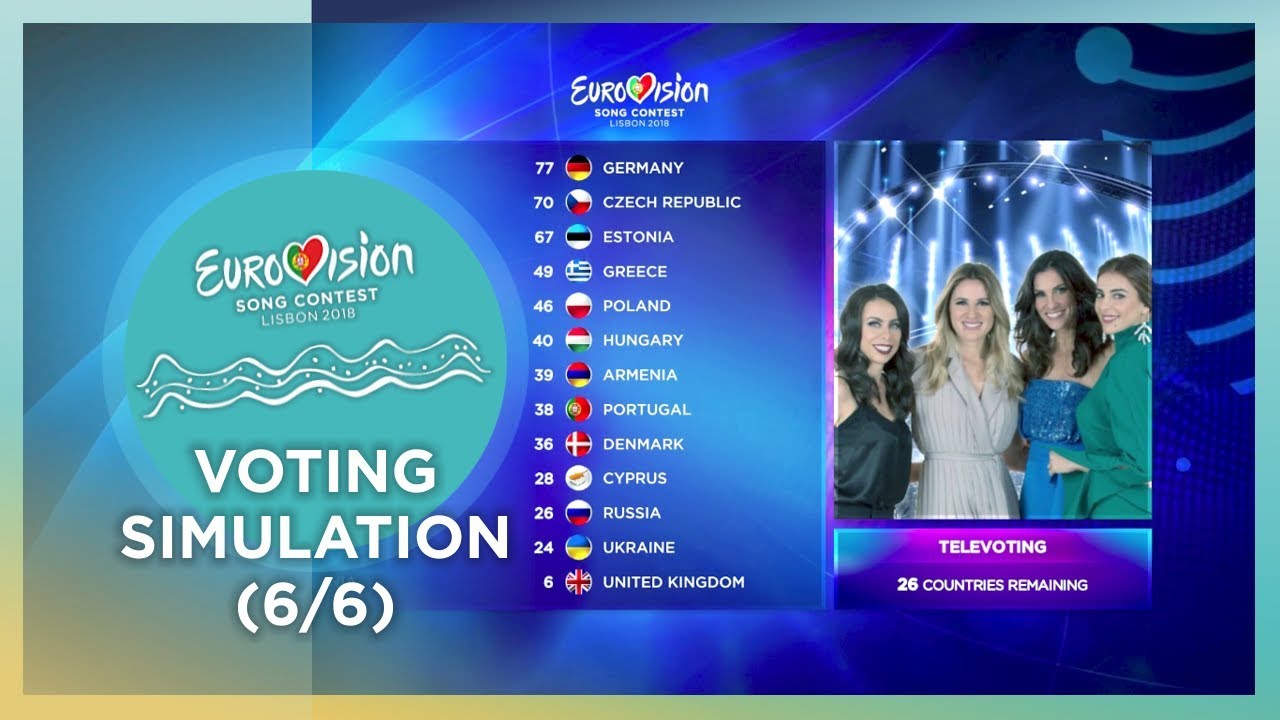The image is a high-definition TV advertisement for the Eurovision Song Contest Lisbon 2018, featuring a detailed ranking of approximately 15 different teams from various countries. The rankings are listed centrally with Germany, Czech Republic, Estonia, and Greece among the top. The title "Eurovision Song Contest" appears prominently in white lettering above the rankings, accompanied by a heart icon filled with green on the left and red on the right. The left side of the image prominently displays "Voting Simulation 6 of 6" and "Eurovision Song Contest Lisbon 2018", decorated with ocean-like wavy lines. The background is a mix of dark blue with a multi-color border transitioning from green to gold. On the right, four women dressed in elegant dresses pose arm-in-arm, smiling at the camera, against a backdrop of bright stage lights. Below them, the text "Televoting, 26 countries remaining" is displayed.